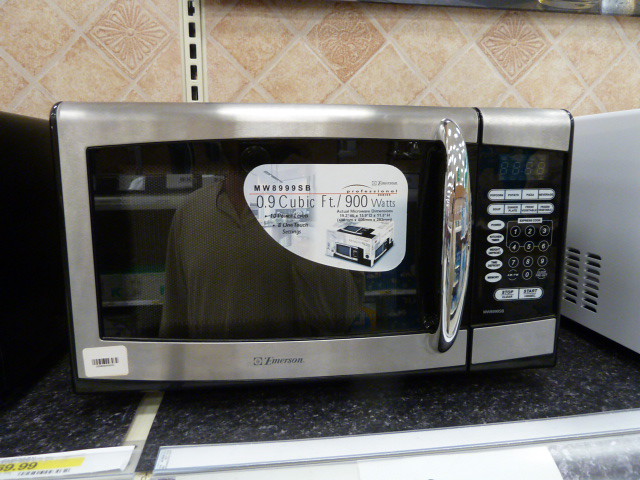This image shows a stainless steel Emerson microwave prominently displayed on a black store shelf, along with a price tag on the bottom left corner that appears to read $49.99. The microwave features a sleek design with a crystal-like, see-through handle on the right side of the door. The central focal point of the microwave is its dark black, tinted window, adorned with a square-shaped white sticker that indicates its capacity and power: 0.9 cubic feet and 900 watts. Surrounding this microwave are other models, including a black microwave on the left and a white one on the right, suggesting this is a section devoted to microwave sales. The background consists of a light beige tiled wall with diamond patterns, adding a subtle yet contrasting detail to the setting. This scene appears to be within a home improvement store or a large retail environment similar to Lowe's or Home Depot.